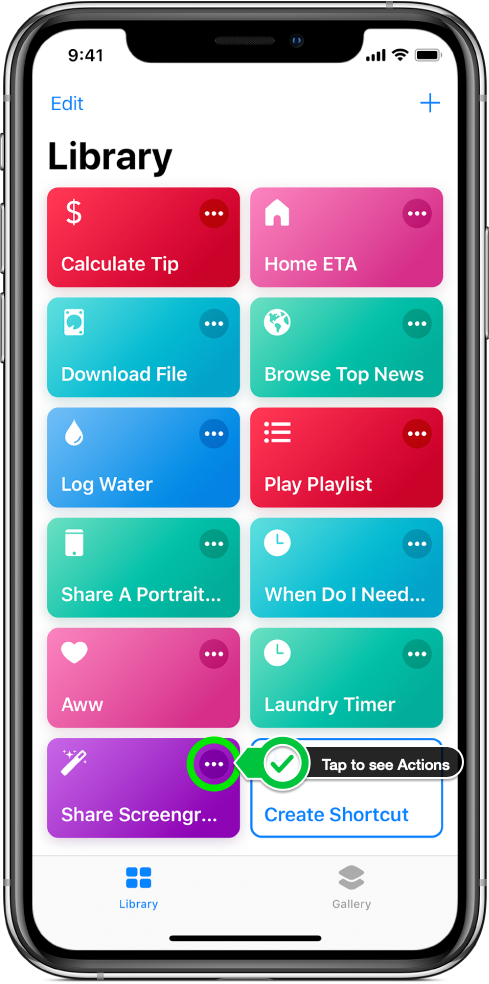Here is a detailed and cleaned-up caption for the described image:

---

The image showcases an Apple iPhone with an app loaded that displays a white background interface. At the top left of the screen, there is a blue "Edit" button while the top right features an "Add" button. Just below these, the word "Library" is displayed in black. The app interface is organized into two columns of tiles, each containing six items.

In the left column, the tiles are listed in descending order as:
1. "Calculate Tip"
2. "Download File"
3. "Log Water"
4. "Share a Portrait"
5. "All AWW"
6. "Share Screen" (appearing as Screen Grabber or Screen Graph)

The "Share Screen" tile is highlighted with a circle around the three dots located in its upper right corner, with a prompt reading "Tap to see actions."

In the right column, the visible tiles are:
1. "Home ETA"
2. "Browse Top News"
3. "Play Playlist"
4. "When Do I Need" (the full title may be hidden)
5. "Laundry Timer"
6. "Create Shortcut" icon

At the bottom of the screen, two menu options labeled "Library" and "Gallery" can be seen.

---

This descriptive caption provides a clear and organized overview of the image, detailing both the layout and content in a structured manner.